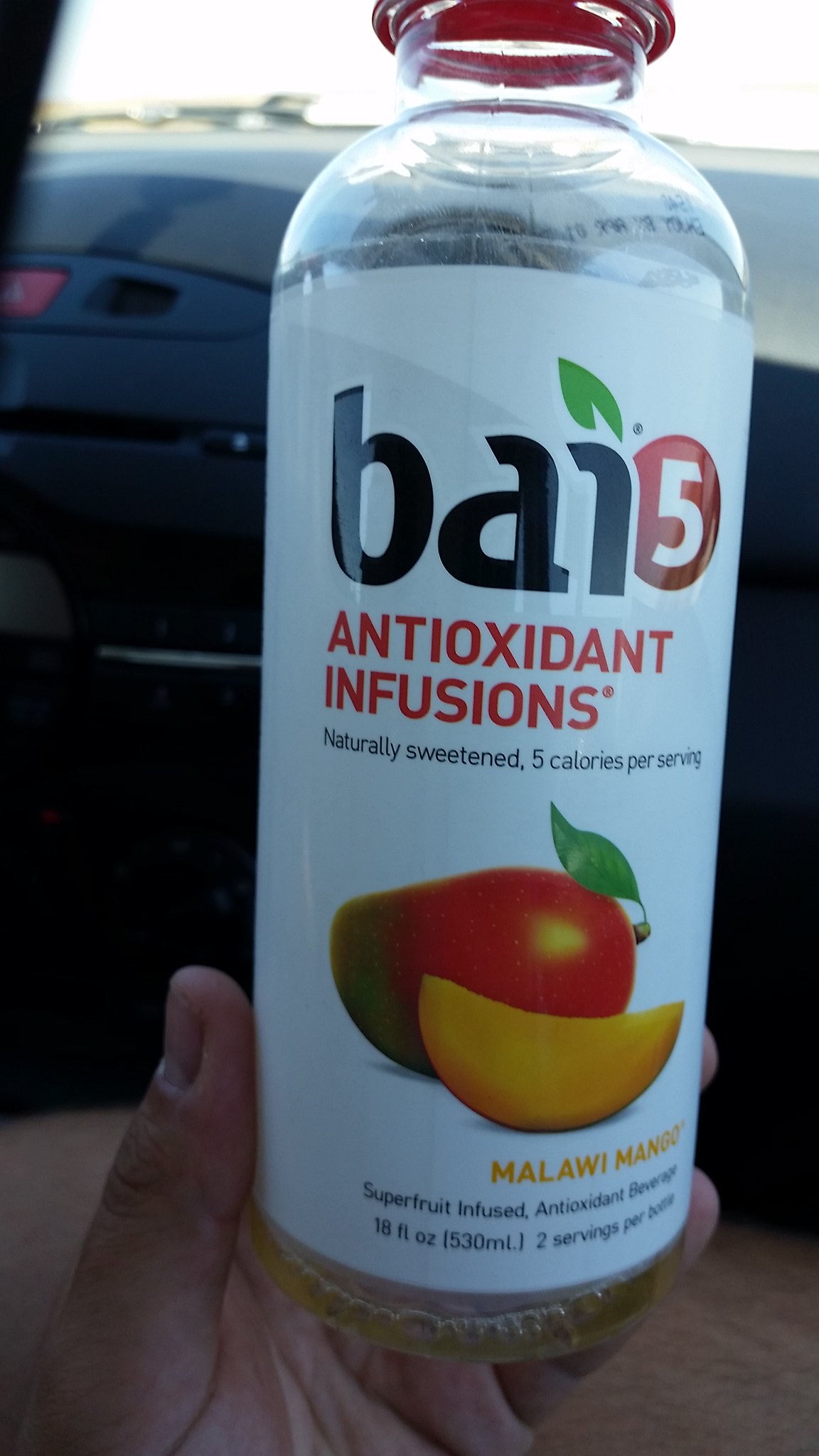In the image, a person is seated inside a car, and you can see their hand holding a clear plastic bottle with a red screw cap and a white label. The label, predominantly white with black text and some colored details, prominently displays the brand "BAI," with the 'I' cleverly dotted by a green leaf. A red circle with a '5' inside indicates the branding of "Bay 5 antioxidant infusions." The label also specifies that the drink is naturally sweetened and contains only 5 calories per serving. There are vibrant images of mangoes on the label - a whole mango with a green leaf and a sliced piece, illustrating the "Malawi Mango" flavor. The bottle contains 18 fluid ounces (two servings), and the liquid inside appears to be yellow. The photo captures a portion of the car's interior, including a black dashboard and likely a glove box, suggesting that the picture was taken in a well-lit environment with some sunlight streaming through the windshield. The person's thumb, palm, and pinky finger are visible, framing the bottle centrally in the image.